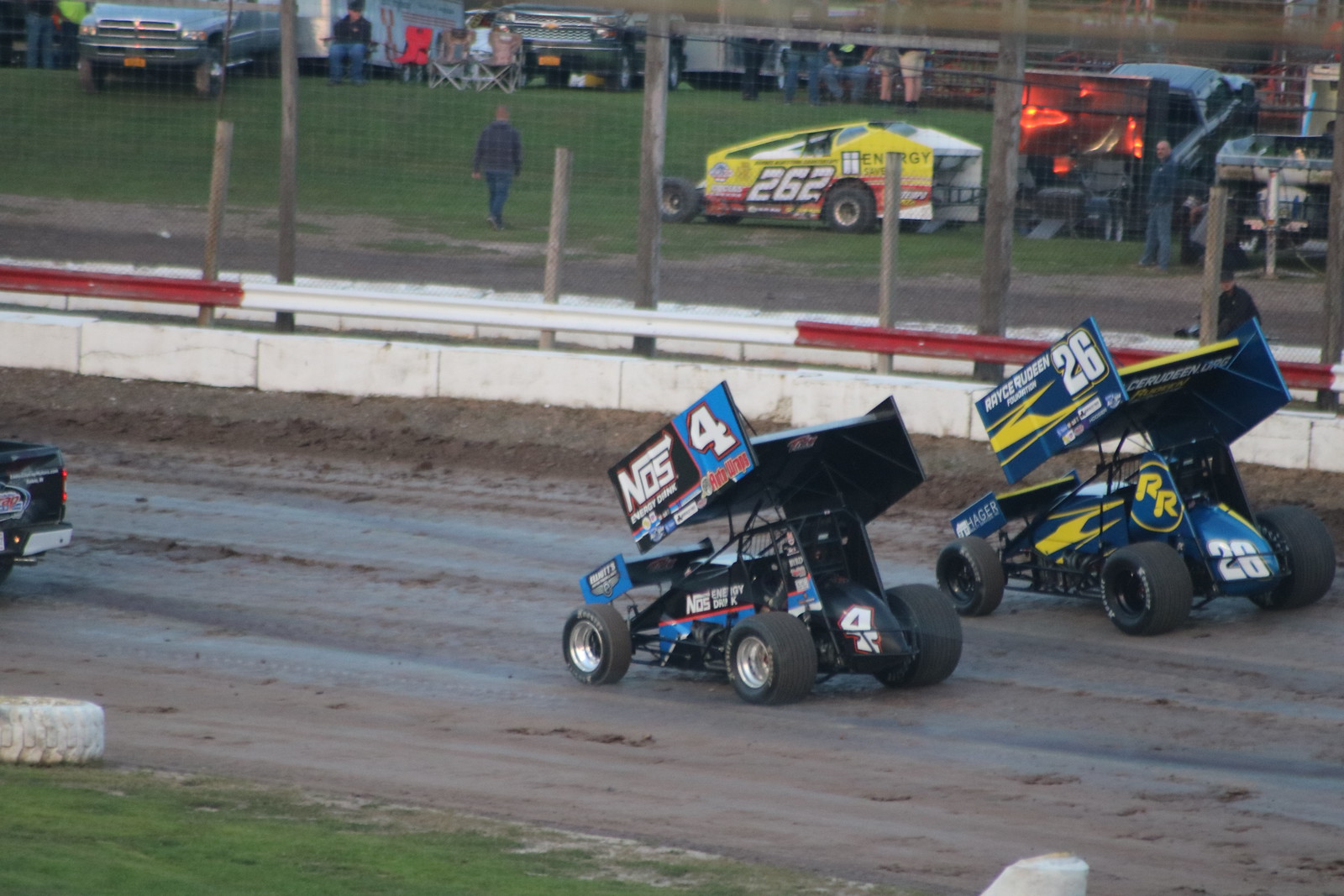In this outdoor photograph captured on a sunny day, the lower right quadrant features two remote control race cars on a mud track. The car on the left sports a NOS logo and the number 4, while the car on the right is marked with the number 26 and branded "Race Routine." These cars, equipped with a hydraulic lifting mechanism, are relatively small and appear to be without drivers. On the far side of the track, a white cement barrier with a red and white guardrail separates the racing area from the grassy field beyond. A cattle fence with wooden posts delineates the boundary, behind which people are seen tailgating, lounging in lawn chairs, and walking around near their parked cars. In the background, a larger yellow vehicle, reminiscent of a cyber truck, bears the number 262. A man in a gray shirt is visible walking near this vehicle, adding to the lively atmosphere of the gathering.